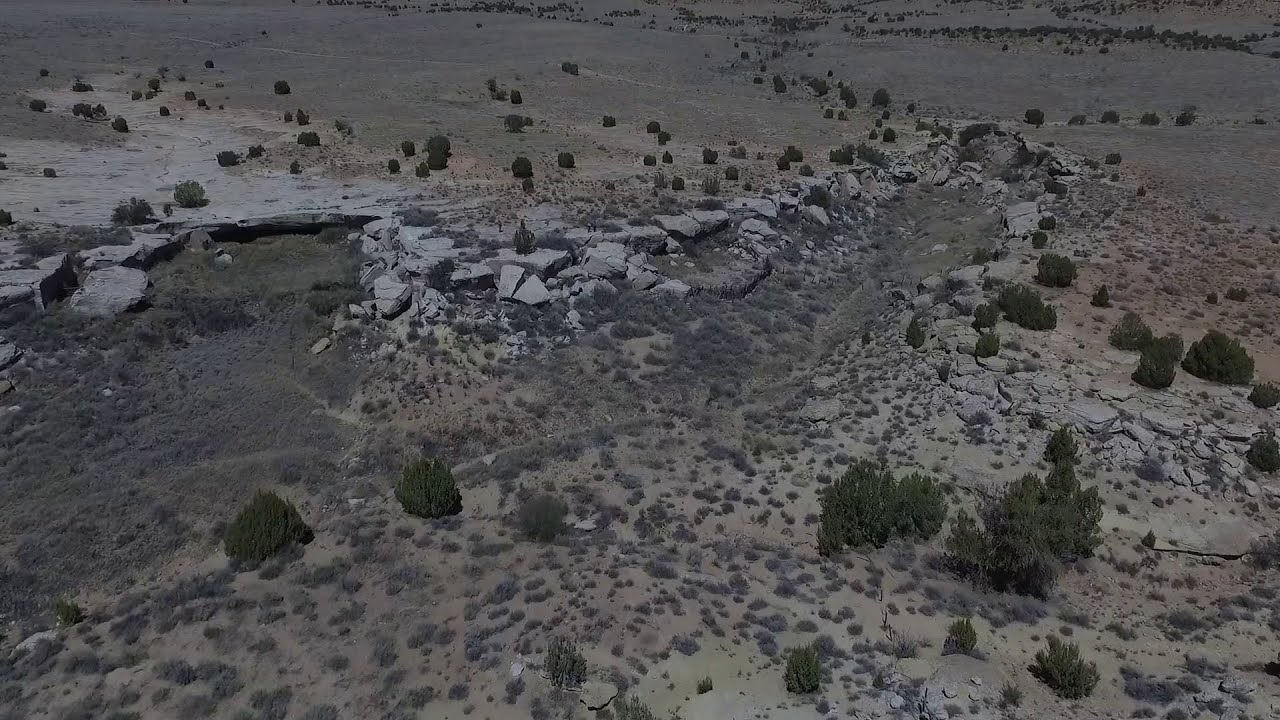This aerial image taken from a drone or flying vehicle captures a desolate, dry landscape, likely a desert or a sparsely vegetated area on the outskirts of a town. The ground is predominantly covered in dirt and sand, with scattered green trees and bushes that occasionally grow tall enough to resemble small trees. Prominently visible are numerous light gray rocks and slabs, broken into rough, uneven pieces that litter the terrain. These rocks surround a noticeable depression in the earth, suggesting a drainage basin or divot where water might pool during rainfall. The overall scene is illuminated by daylight, revealing the earth's stark, grayish cast interspersed with sparse vegetation, giving the land a barren, arid appearance.